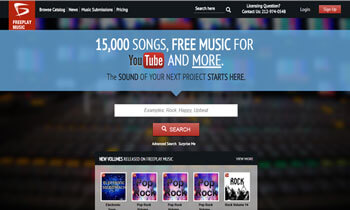This is a landscape-format, color screenshot of a website displayed on a computer screen. The website appears to be branded as "Free Play Music." At the top of the website, there are four tabs labeled: "Browse," "Gaming," "News," "Music Submissions," and a somewhat blurred tab that might read "Pricing." 

In the middle of the top section, there is a search bar labeled "Search here," allowing users to type in song titles of interest. To the right of the search bar is a section labeled "Questions," providing a phone number for inquiries.

The central message on the page reads, "15,000 songs, free music for YouTube and more. The sound of your next project starts here," displayed prominently across a blue banner. Below this, there is a search button for users to look for specific music.

Further down the page, users can see new volumes of music available, showcasing various albums and individual songs. The background of the website is predominantly dark and blackish, providing a contrasting backdrop to the blue banner and featured content.